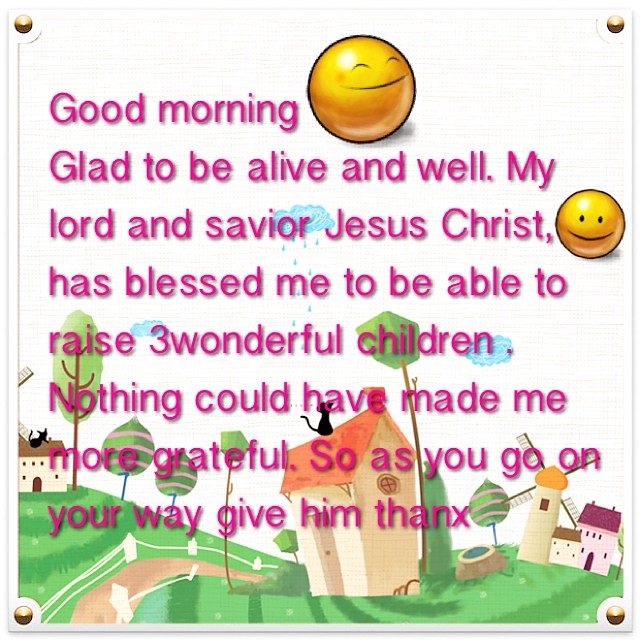The image depicts a white plaque with a slightly rough texture featuring an inspirational message in pink and purple fonts. At the top of the plaque, an orange smiley face ball with a glow surrounding it is positioned, radiating a welcoming vibe. The text reads: "Good morning, glad to be alive and well. My Lord and Savior Jesus Christ has blessed me to be able to raise three wonderful children. Nothing could have made me more grateful. So as you go on your way, give him thanks." On the right side of the plaque, another smiley face ball with two black dots for eyes and a slim line for a mouth faces forward.

The background of the plaque includes a whimsical cartoon scene with several elements. In the center, there is a slightly tilted house with an orange stove roof and a light brown walkway lined with a rope barrier. This house is flanked by two other houses, each adorned with black cats on their roofs. On the bottom right corner, there is a windmill adjacent to a pink house with a purple roof, and a green tree with light pink stripes stands nearby. The sky features white and blue cartoonish clouds with a hint of rain, further enhancing the playful atmosphere of the scene.